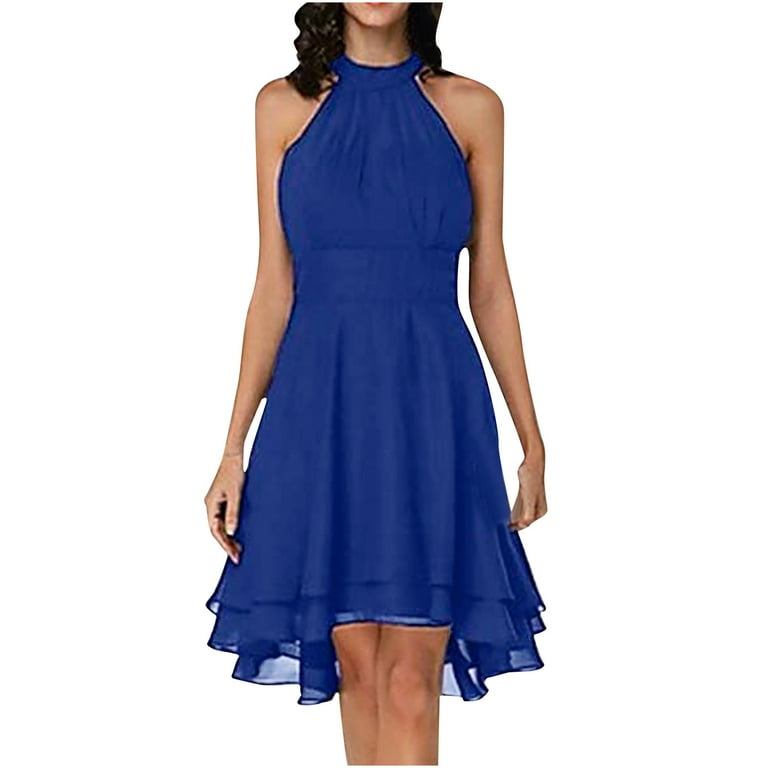This vertical image features a young woman, cropped so that only her lower face to just below her knees are visible. She is dressed in an elegant, dark blue party dress, characterized by a sleeveless design and a high neck collar with a blue strip wrapping around. The dress has a fitted waist, accentuating her figure, and features a dual-layered skirt: a shorter, solid inner layer and a longer, mesh outer layer that offers a delicate, slightly see-through quality. The dress is shorter in the front, stopping just above her knees, and extends longer on the sides. The woman's long, dark brunette hair falls to her shoulders, framing the visible part of her face and neck. Her arms rest at her sides, with her left leg positioned behind her right. Some parts of her body, including her knees and hands, appear oddly altered, hinting at possible digital manipulation. Despite these anomalies, the dress appears well-fitted and stylish, perhaps suggesting that she is modeling the garment.